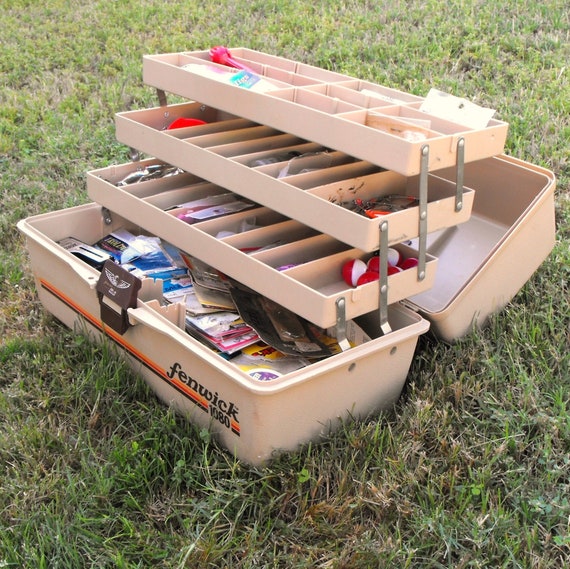This detailed close-up photograph captures an open tackle box positioned on short, green, and wheat-colored grass. The tackle box, which is tan in color, is fully opened with its top lid lying back onto the grass, revealing its interior. The inside of the lid shows three vertically stacked shelves that unfold over each other from the bottom of the box. Prominently featured on the front center of the box is an orange horizontal line with a black horizontal line beneath it, and the brand name "Fenwick" displayed in black on the top right side of the orange line. Within one of the small compartments on the shelves, a collection of red and white fishing bobbers is visible. Each of the shelves contains various compartments. At the bottom of the box, there are several items still in their packaging, though the specific contents are indiscernible.